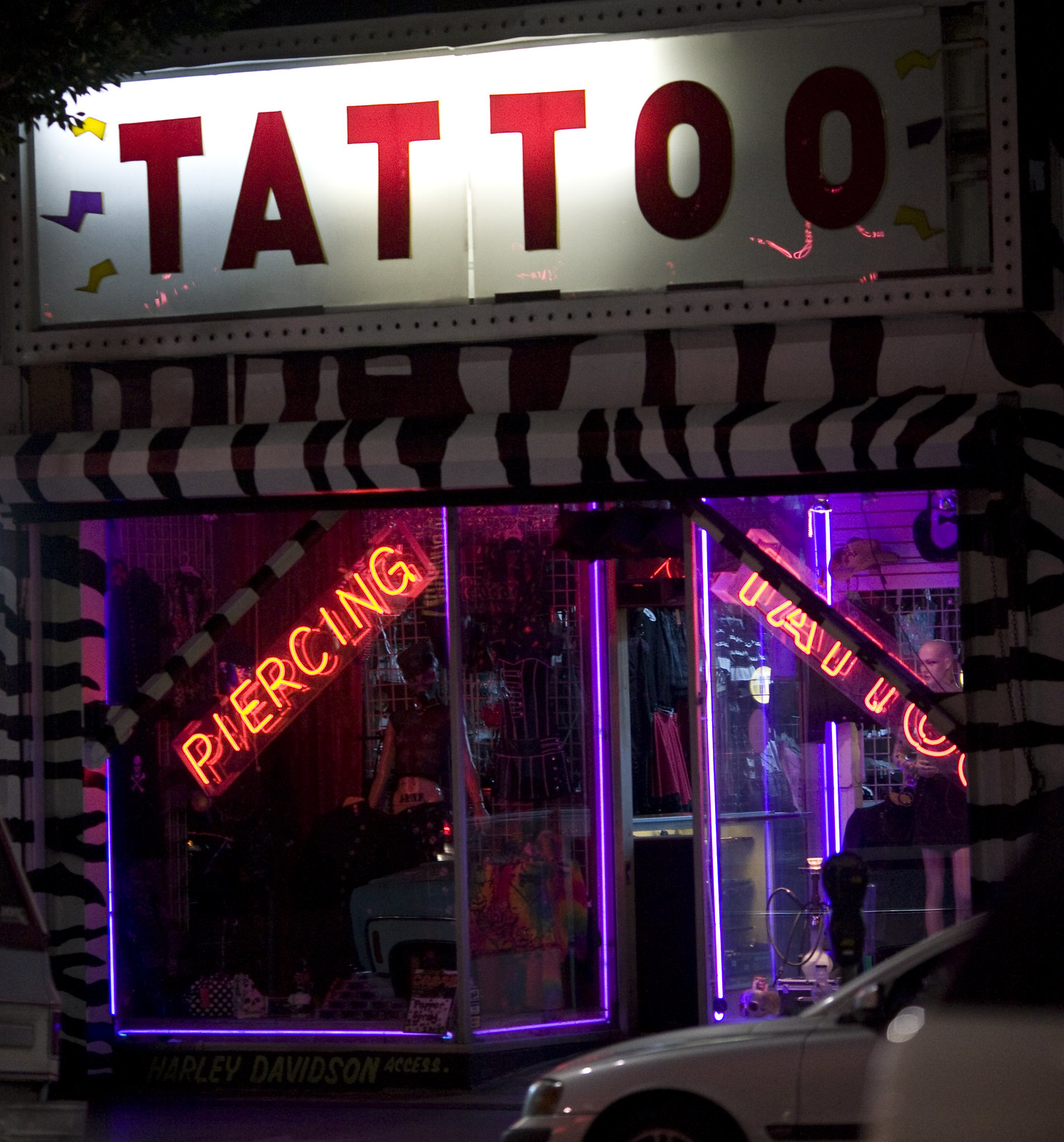This nighttime photograph captures the storefront of a tattoo parlor. Dominating the scene is a large white sign with red letters reading "Tattoo." Below this sign, the exterior features a striking zebra stripe design that spans above and around the windows. The storefront is bordered by vivid purple neon lights, creating a glowing frame around two large windows. The left window has an angled neon sign in yellow-orange that reads "Piercing," while the right window displays a red neon sign saying "Tattoo." The windows reveal mannequins inside, though it's too dark to discern their attire clearly. Between the windows is an open door. Outside, partially visible in the lower right corner of the frame, the front end of a white car faces left. The overall scene exudes an inviting yet mysterious ambiance, typical of an establishment caught at night.